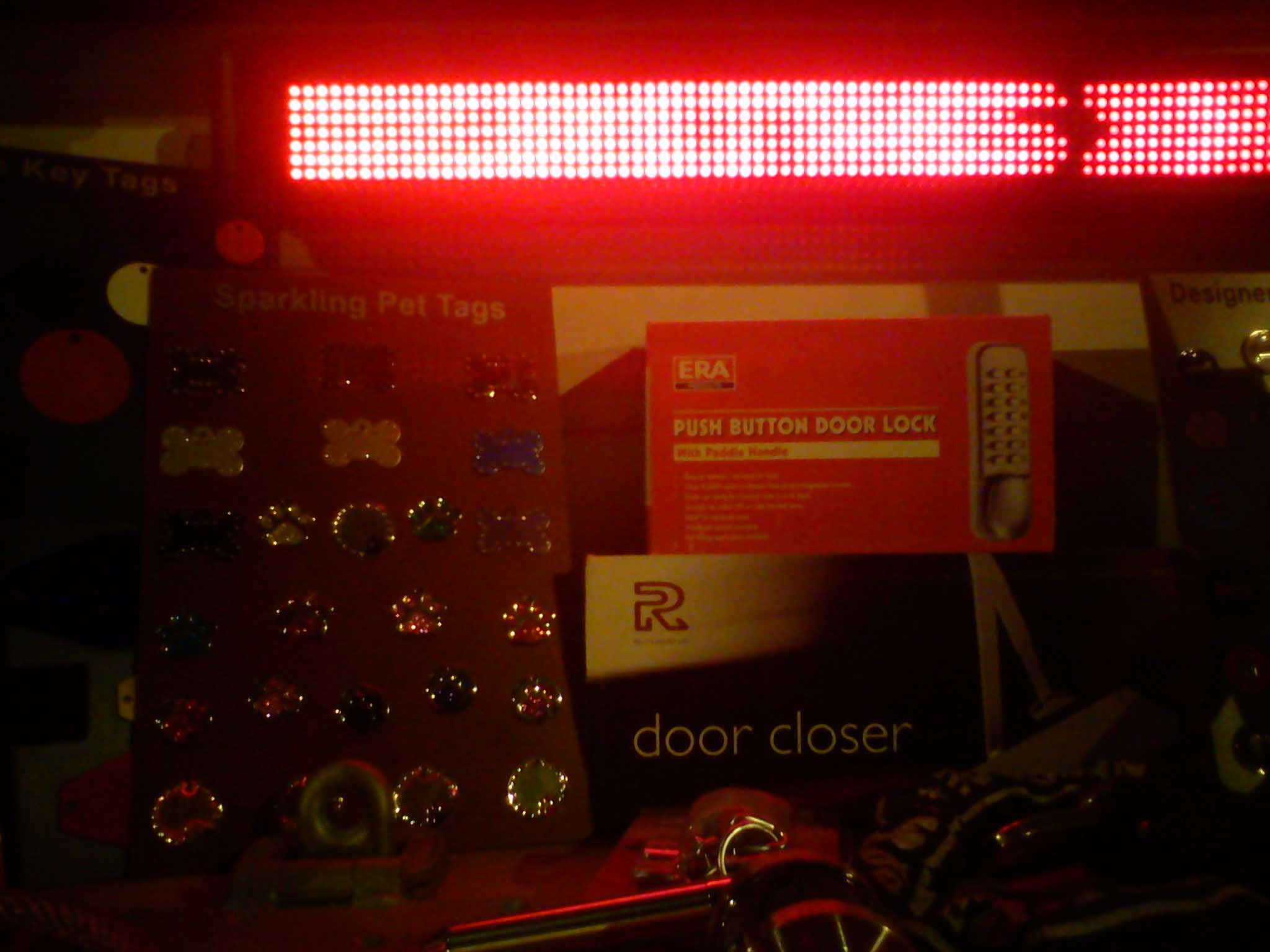The image depicts a display illuminated by small pin-sized red lights at the top, casting a red glow over the scene. At the center, prominently featured, are various sparkling pet tags, some designed in the shape of paws and dog bones, with a glass or jewel-like appearance. These tags are arranged on an upward-standing red surface. Adjacent to the display, on the right, is a boxed item labeled "push-button door lock," resembling a tan remote control, and another box indicating a "door closer." The overall composition includes miscellaneous items spread out on the table underneath. The image is somewhat dark, suggesting a mishmash of items, perhaps in a shop or a cluttered space, with contrasting bright neon lights and colorful labels adding to the visual complexity.